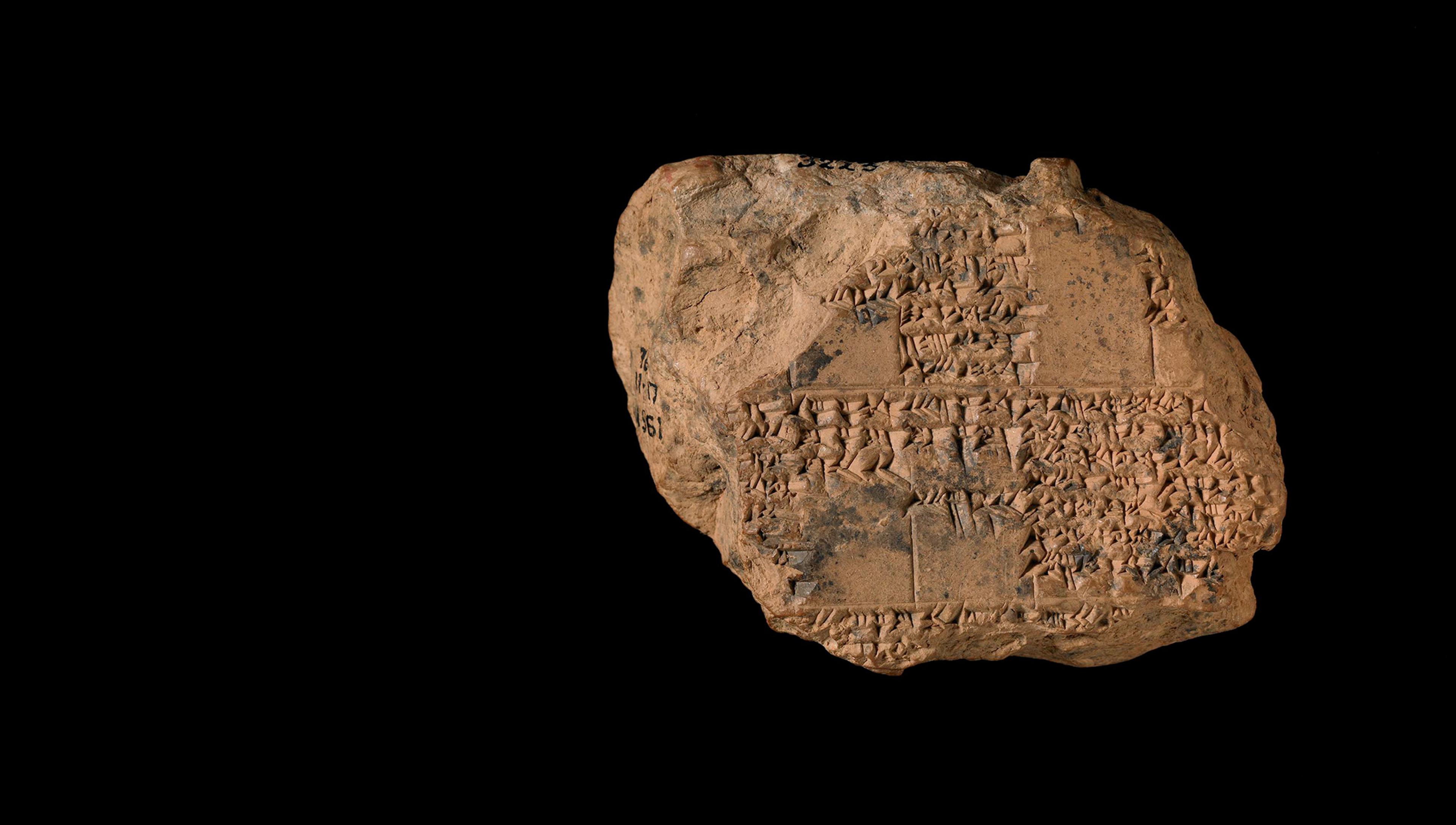The image showcases a wide-angled photograph of a carved stone artifact set against a matte black background, giving it a stark contrast. The artifact, likely ceramic or hardened clay, is a roughly parallelogram-shaped piece with slanted sides and a mostly straight top and bottom, though it is heavily worn and chipped, especially in the top left corner. The stone's color varies from light clay to darker brown, with hints of gray. Intricate carvings cover its surface, depicting detailed patterns that might include hieroglyphics or human figures, though the exact imagery is not entirely clear. There are also what appear to be sharpie marks and text, including discernible numbers like "7," "11.17," and "1961," indicating its cataloging as a museum artifact. This piece is positioned slightly to the right within the frame, and the overall composition and details suggest its historical significance.